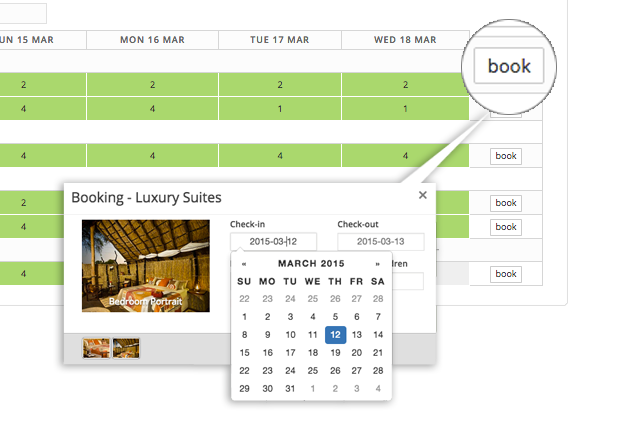The image depicts a detailed booking system for luxury suites, potentially aimed at a high-end vacation resort. At the top, there is a header indicating dates from Sunday, March 15th, to Wednesday, March 18th. Each date is followed by columns filled with data points, typically marked in green rows, each indicating availability or specific booking details, numbered as "2 2 2 2."

On the right side, there is a prominent column titled "Book in a Box," featuring what appears to be a magnified section of the information for clarity. Below this, a dialogue box labeled "Booking Luxury Suites" includes two portrait pictures, presumably of the suites being offered. 

At the bottom left of the image, there is a check-in and check-out feature powered by Google, currently set to March 12th, 2015, for check-in, and the next day for check-out. 

The suite itself is pictured in a separate section, depicting a hut-like structure with a slanted roof supported by a pole. The roof appears to be made of hay, held together by horizontal bamboo strips, set against a visible sky. 

Below Sunday, March 15th, each green row, marked as "2 2 2 2," continues through the following columns, suggesting various data points critical to the booking process. Each row is equipped with an option to proceed with the booking, covering all four days up to Wednesday, March 18th.